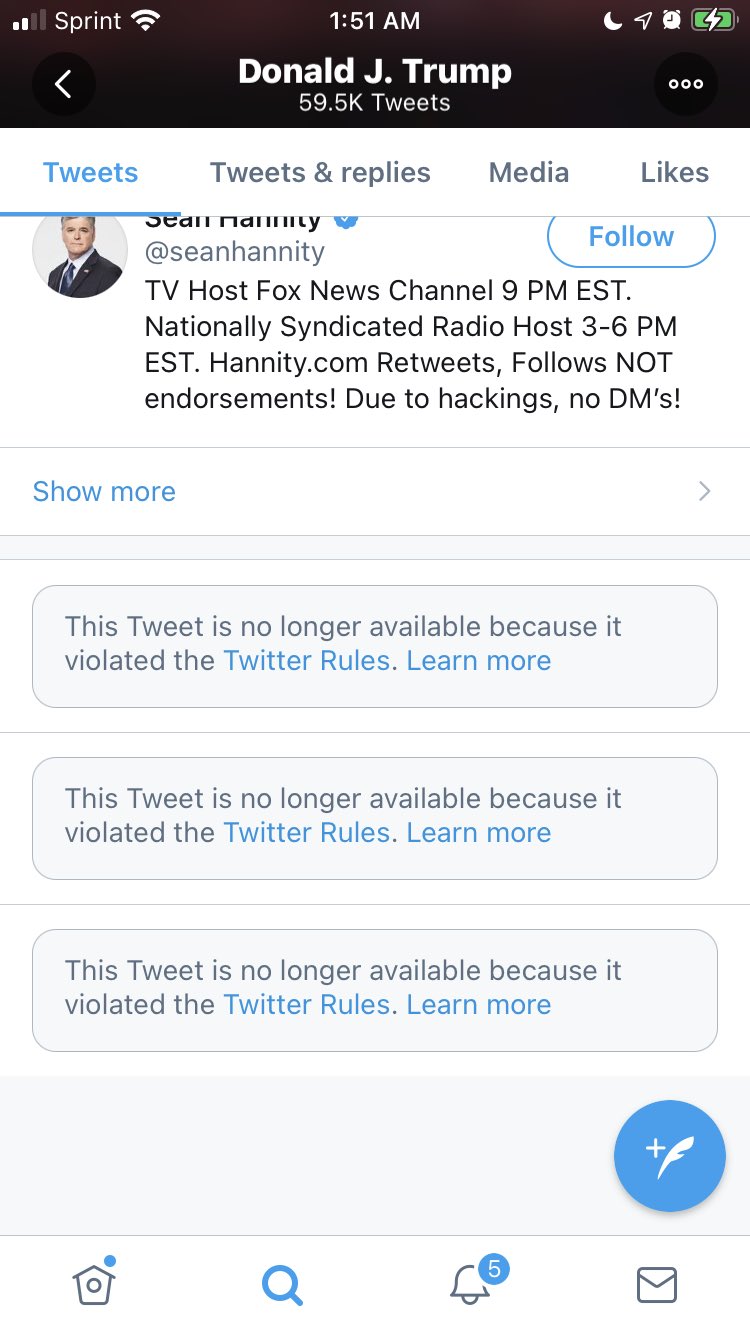Title: A Glimpse into an Active Twitter Page

Caption: Taken at 1:51 a.m. with a Sprint signal showing two out of four bars and a fully charged battery, this screenshot captures the enigmatic Twitter profile of Donald J. Trump. The image shows his impressive tweet count of 59.9 thousand and reveals a series of notifications, represented by a blue bell icon with the number five inside a circle. Prominently featured is a tweet interaction with Sean Hannity, the noted Fox News host and nationally syndicated radio presenter. Hannity’s handle, @SeanHannity, stands out along with his broadcasting schedule—9 p.m. EST on Fox News Channel and 3 to 6 p.m. EST on his radio show. Due to previous account hackings, Hannity’s profile discreetly notes "retweets follows not endorsements," and he mentions he doesn’t engage in direct messaging (DMs). Interestingly, multiple notifications indicate several tweets have been removed for violating Twitter's community guidelines. The UI elements, including a blue mailbox icon with a white plus and feather, hint at Twitter’s functionalities. This detailed glimpse illustrates the interaction dynamics and vigilant moderation within the Twitter environment.